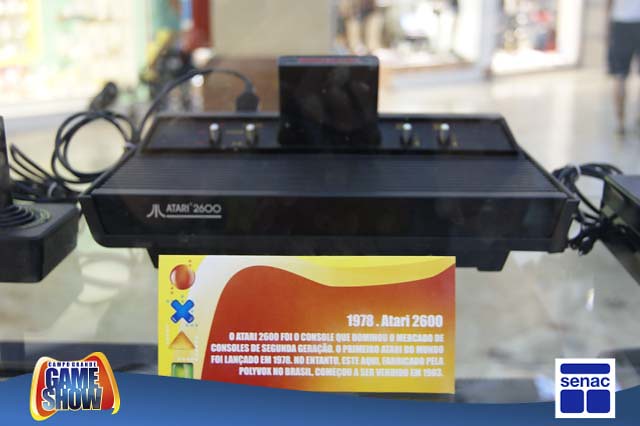This image features a vintage 1978 Atari 2600 gaming system prominently displayed against a blue background. The black rectangular console showcases four silver levers on the back and an upright black cartridge in the center. The front left side features the Atari logo and "Atari 2600" label. The console is set atop a white or marble table, sharing the space with a joystick controller on the left and coiled black wires. There's a partial view of another black device with more coiled wires to the right.

In front of the Atari is a large, orange and yellow display card with cartoonish controller buttons on the left side. This card includes the Atari's identification, reading "1978 Atari 2600," along with additional information in what appears to be multiple languages, possibly Spanish or Portuguese. The card seems to indicate the console is part of an exhibition, reinforcing the museum-like atmosphere. 

Logos for "Game Show," marked with a cartoonish controller, and "CENAC" (or "SCNAC") in blue letters, appear in the bottom corners of the image. The background reveals a well-lit, open-space retail or museum area with people and displays visible, suggesting a public exhibit setting.